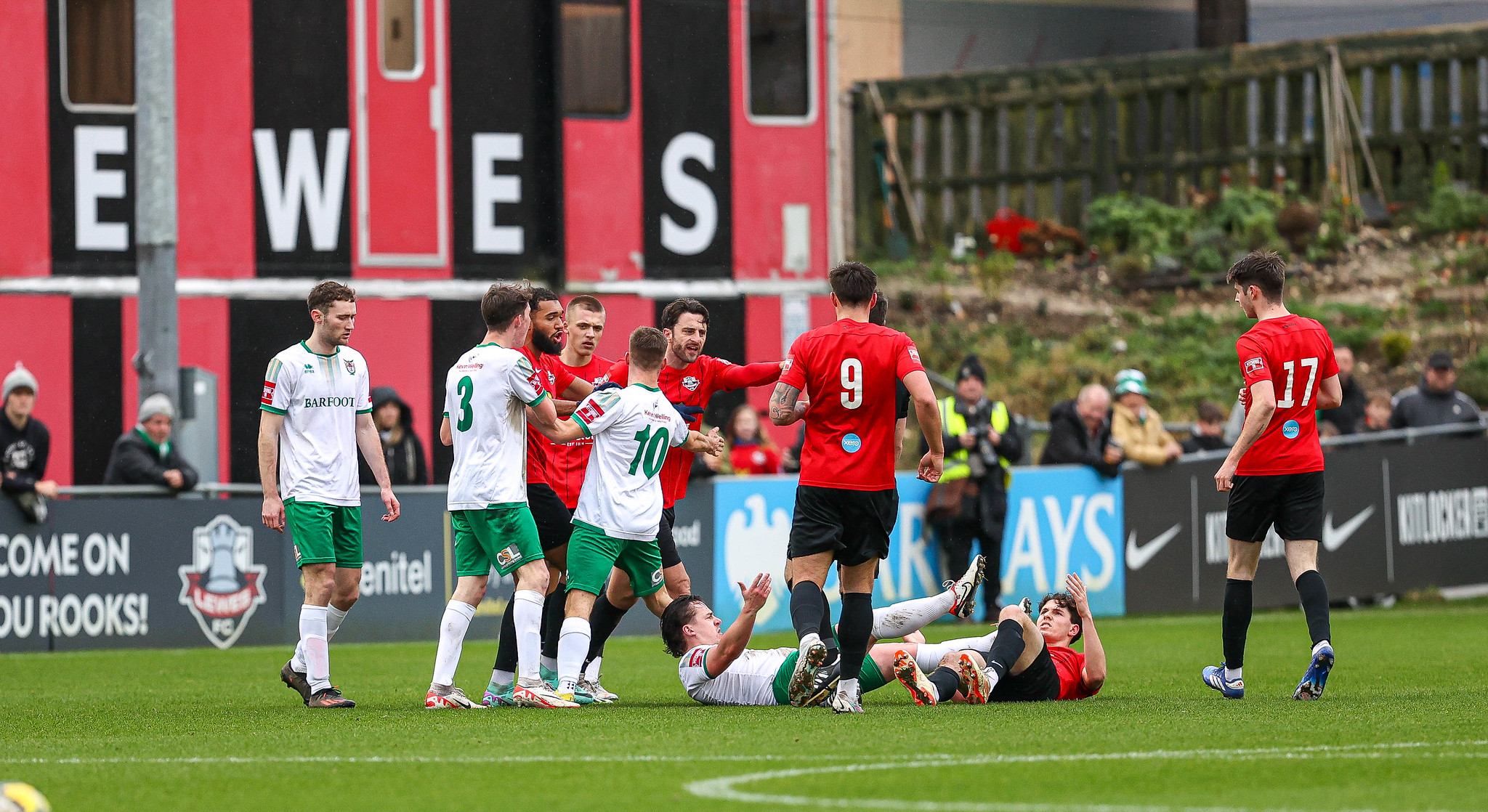The photograph captures an intense moment in a lower league English football match, likely identified by the presence of familiar advertisements such as Barclays Bank and a banner that reads "Come On You Rooks." The professionally framed and clear image shows a scuffle on the pitch, where one player from the red-shirted team with black shorts and black socks, and another from the white-shirted team with green shorts and white socks have collided and fallen to the ground. This collision has seemingly sparked tension as several players, with arms spread aggressively, appear to either engage in or try to diffuse the conflict. The bright green grass field contrasts with the colorful uniforms, and in the background, a sparse crowd near the pitch boundary is seen separated by hoardings displaying various advertisements, including the Barclays Bank logo and Nike symbols. Despite the altercation on the field, the day appears clear and free of adverse weather, highlighting the vivid colors and dynamic scene of the match momentarily halted by the dispute.